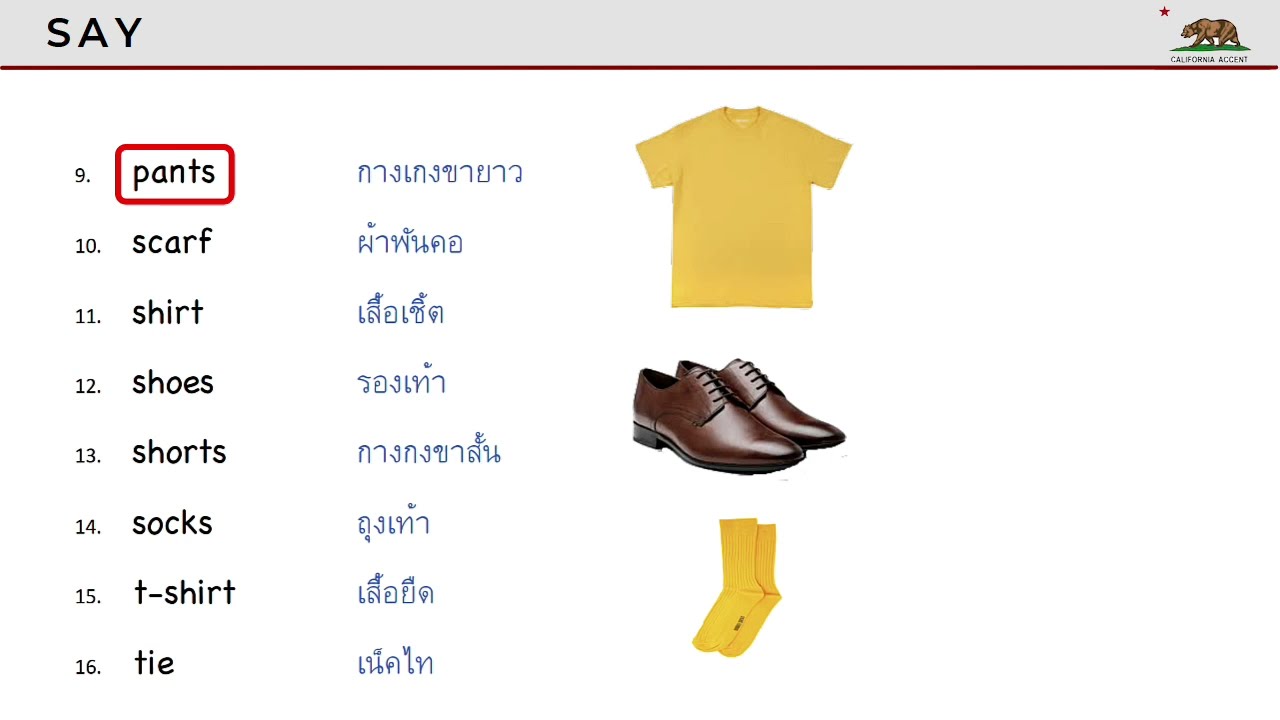This image is a snapshot of a webpage from California Accent, featuring a white background. At the top, there's a gray rectangular banner that includes the California state flag with a brown bear on grass and a red star in the upper left corner. To the left of the bear, the word "SAY" is prominently displayed in black, all-caps text with a red underline. Below the banner, the webpage title "California Accent" is visible.

On the left side of the image, there are numbers 9 through 16 listed vertically. Each number corresponds to a different clothing item: pants (9), scarf (10), shirt (11), shoes (12), shorts (13), socks (14), t-shirt (15), and tie (16). To the right of each English word, there are blue symbols, presumably translations in another language.

To the right of this list, there are three photographs: at the top, a gold short-sleeved t-shirt; in the middle, a pair of brown (or black-brown) dress shoes; and at the bottom, a pair of gold or yellowish ankle socks. The overall layout resembles a PowerPoint slide with clear sections and visuals for easy comprehension.